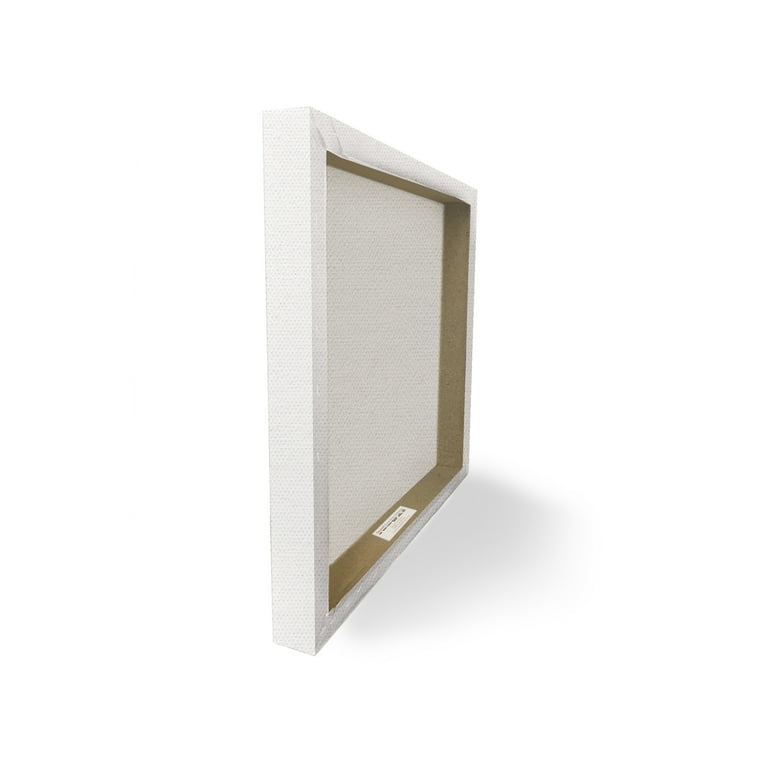This image is a detailed and realistic color photograph of the back of a square-wrapped canvas frame. The canvas is oriented in portrait mode and positioned at a three-quarter angle, standing on its edge. The front of the canvas is facing away from the camera, revealing the light wooden frame and the interior back side of the canvas. The white canvas is tightly wrapped around the wooden rectangular frame, which is stapled and glued at the edges. There is a small white sticker with illegible writing on the bottom center of the stretcher stick. The canvas is isolated on a pristine white background, casting a very light shadow to the right, suggesting that the light source is coming from the upper left. The overall composition lends a photographic representational realism to the image, capturing the intricate details and textures of the canvas and frame.